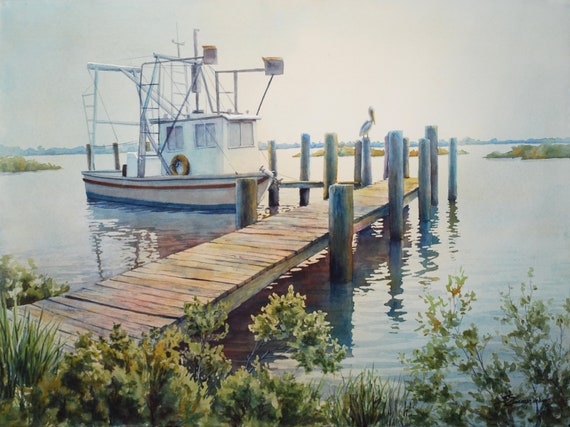In this detailed landscape-oriented watercolor image, we see a serene waterway, likely a large river or an ocean, with various elements coming together to create a peaceful scene. Centered prominently is a white boat adorned with red and blue stripes, equipped with rails, ladders, and a tan-colored life float on its side. The boat is docked at a wooden pier that stretches diagonally from the bottom left to the top right, stopping at the water. The dock, featuring uneven, mildew-covered posts with some hues of green and white, is also flanked by reedy, swampy vegetation in shades of dark green and yellow. 

A pelican perches calmly on one of the dock's posts, adding life to the scene. The background from the top left to the top right corner transitions into a grayish sky, suggesting a bright but overcast spring or summer day. In the mid-ground, small islands with patches of yellow punctuate the water, providing a sense of depth and distance. The water itself is a tranquil blue, mirroring the sky's muted tones and the surrounding greenery, creating an overall cohesive and calming composition. Notably, the picture lacks any human presence or text, allowing the natural setting to be the central focus.